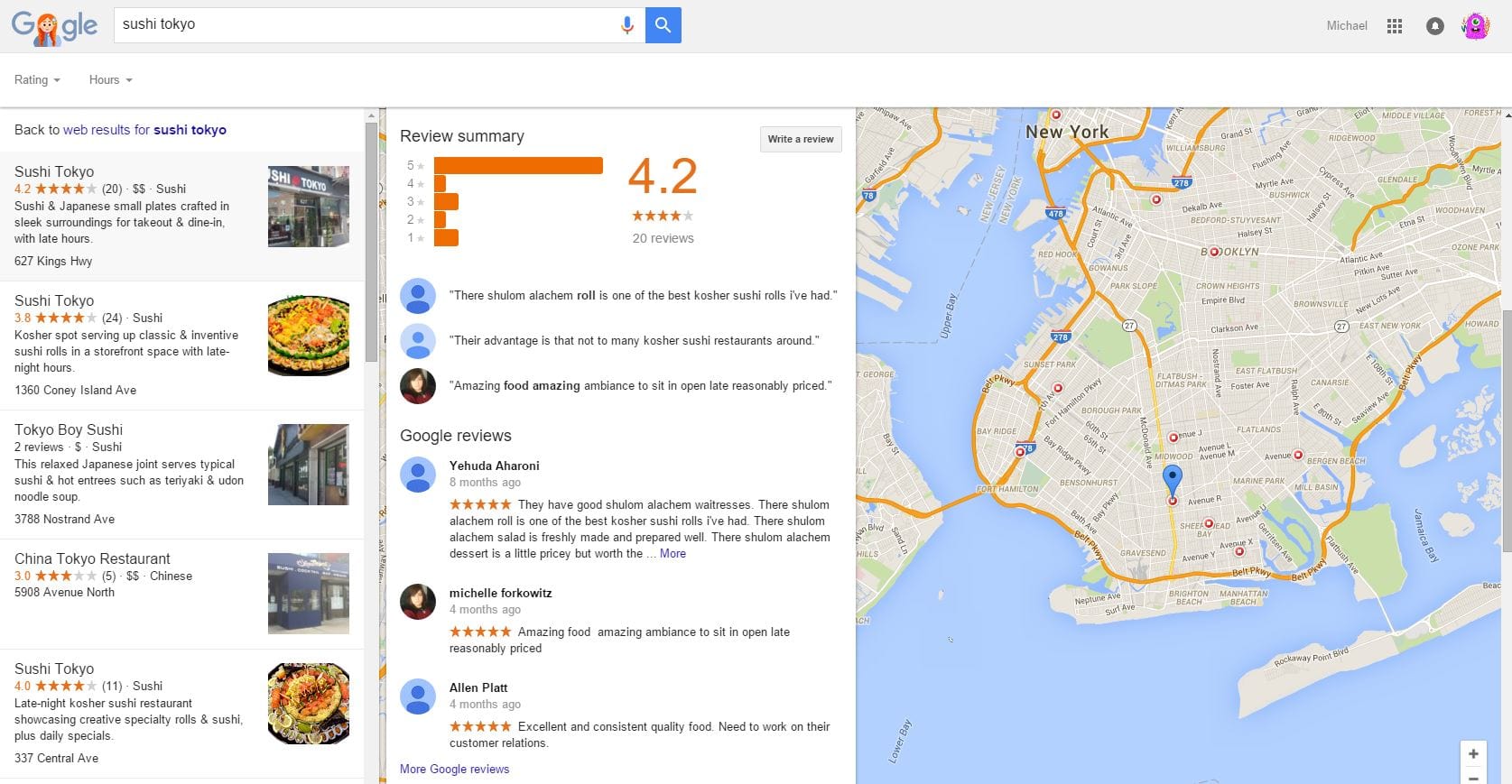In this screenshot set against a white background, the focal point is a Google search bar located in the upper left corner. The Google logo is creatively illustrated with a young girl replacing the two O's. Below are dropdown options for ratings and hours. 

The search results displayed include various sushi restaurants. Starting from the left, there is a vertical navigation bar. The primary result is "Sushi Tokyo," boasting a 4.2-star rating, signified by yellow stars, and pricing indicated by two dollar signs. It has garnered 20 reviews and offers sushi and Japanese small plates in a stylish setting for both dine-in and take-out, located at 627 Kings Highway.

The next result is another "Sushi Tokyo," with a 3.8-star rating from 24 reviews. It is described as a kosher spot serving classic and inventive sushi rolls in a storefront space that stays open late. An image to the right shows an appealing large platter of sushi.

Following this is "Tokyo Boy Sushi," although no additional details are provided in this screenshot. Finally, there is "China Tokyo Restaurant," which has a 3-star rating from 5 reviews. It specializes in Chinese cuisine and is situated at 5908 Avenue N.